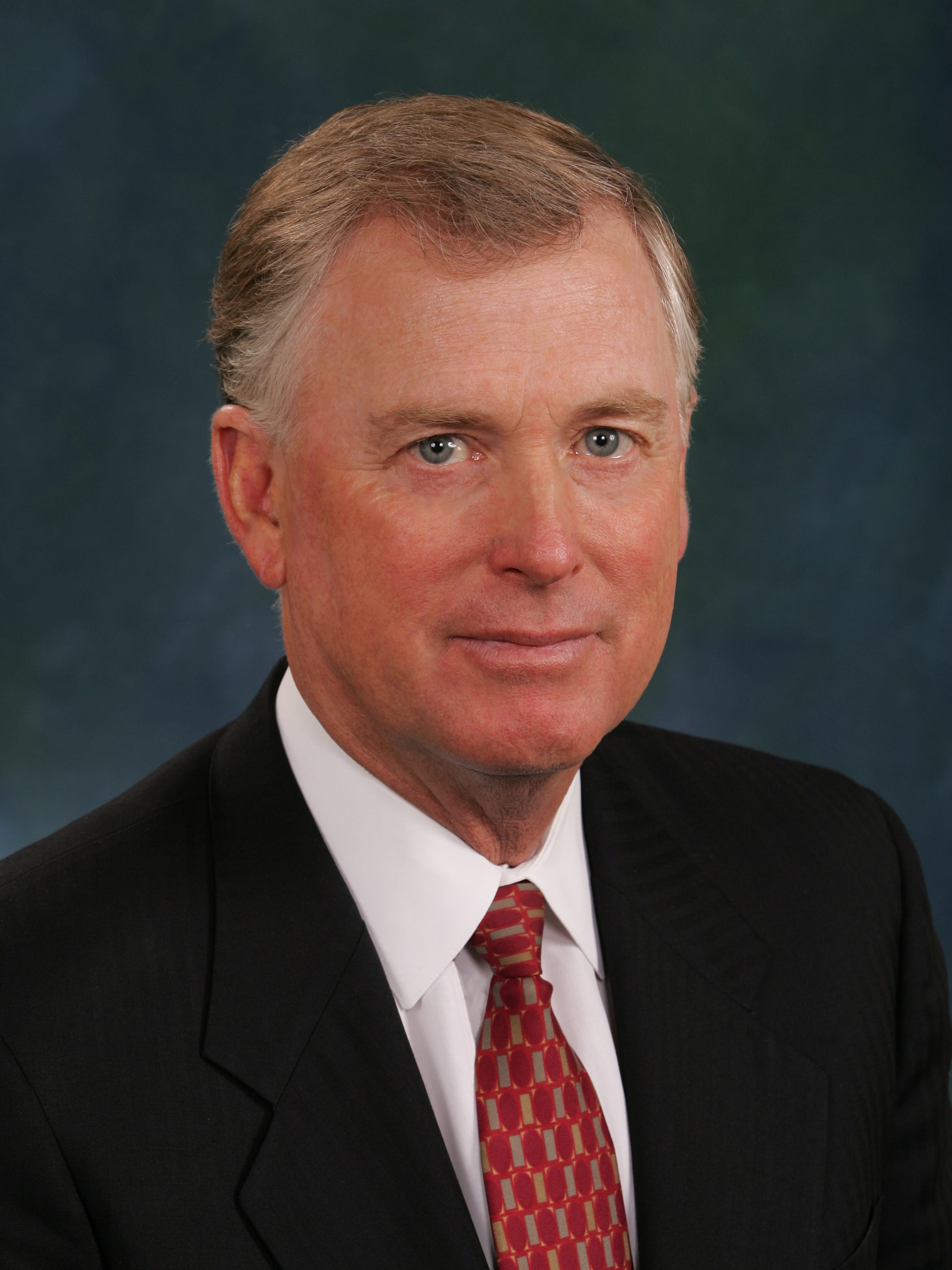This high-resolution professional headshot features Dan Quayle, a politician in his fifties. He is dressed in a formal black suit jacket paired with a white collared button-down shirt. His tie stands out with its red and gray patterned design, prominently featuring more red than gray. Quayle's hair is light brown with noticeable graying on the sides, and he has green eyes. His expression is slightly serious with a very slight smile, not showing any teeth. The background of the photograph is a charcoal gray, which complements the professional and polished appearance of the portrait. The image is cropped closely to show only from the upper torso upwards, capturing the details of his attire and facial features clearly, with his smooth skin adding a refined touch to his seasoned look.